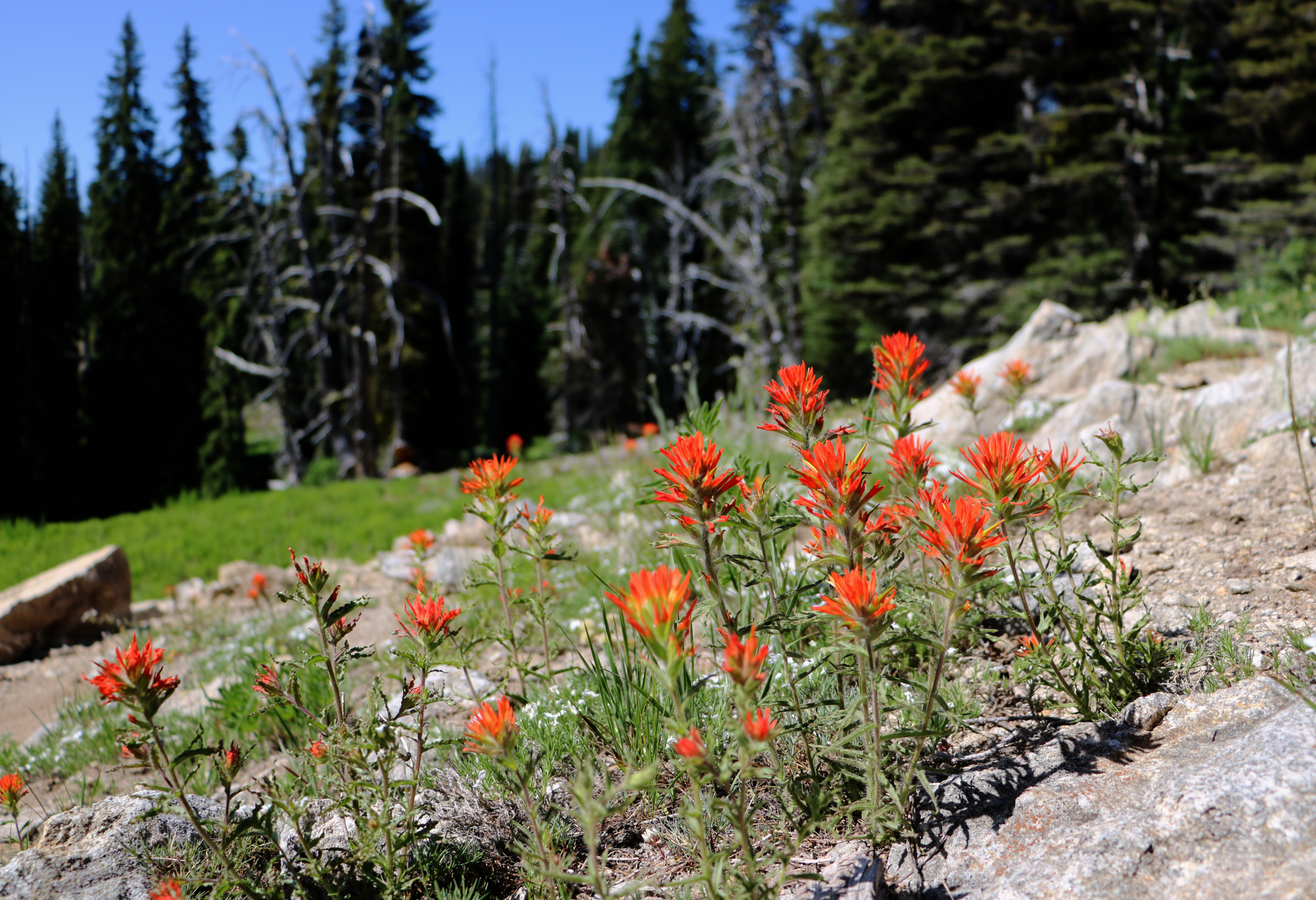A horizontal image captures a rocky hillside adorned with lush, green grass, dotted with exposed rocks and scattered stones. In the background, a dense stand of fir trees frames the scene, their evergreen needles lending a sense of tranquility. Prominently featured in the lower center to middle portion of the image is a cluster of vibrant red wildflowers in full bloom. These wildflowers, with slender green stems and long, thin leaves, boast multiple blossoms ascending along the stalk. Each flower displays a light yellowish base transitioning to a striking orangish-red hue towards the tips, adding a lively splash of color to the verdant landscape.